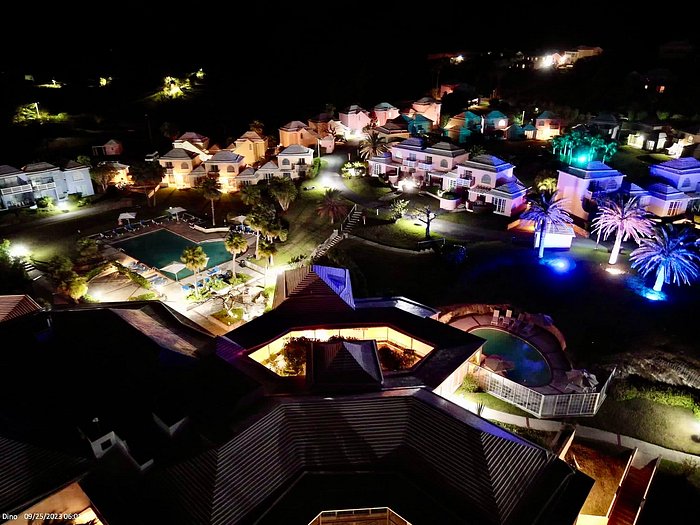The image presents an aerial night view of a luxurious resort community, likely located in Dubai or a similar Middle Eastern region, characterized by its distinctive architecture and abundant palm trees. The scene showcases a sprawling setup of rental villas rather than a single building hotel, indicative of an exclusive, gated neighborhood. On the left side of the image, an L-shaped commercial pool with greenish-blue water is prominently featured, surrounded by three white umbrellas and multiple lounge chairs, giving off a serene, inviting ambiance. Adjacent to the left side, there are several palm trees, both in clusters and individually, enhancing the resort's tropical aesthetic. Towards the middle right of the image, a jacuzzi is visible, encircled by four lounge chairs, two umbrellas, and a white fence, providing a sense of privacy and luxury. The street lights scattered throughout the resort cast a soft glow on the modern, Mediterranean-style villas, highlighting their elegant, light-colored facades.